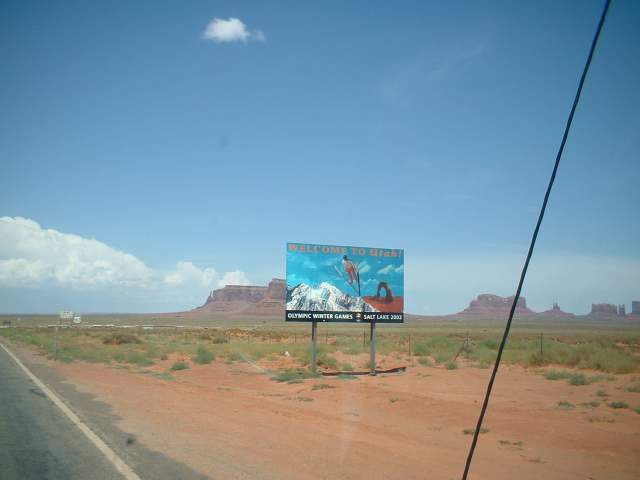The photograph depicts a scenic view along the side of a freeway, primarily focused on a desert landscape. On the left, the edge of a long freeway is visible, stretching into the distance. The right side, where the viewer's attention is drawn, features a barren desert area characterized by reddish soil and sparse clumps of bleached, dry grass. In the background, a series of raised plateaus, which resemble mountains but are not quite as elevated, adds depth to the scene.

The centerpiece of the image is a prominent billboard, advertising the Olympic Winter Games set to be held in Salt Lake in 2024. The billboard's top reads "Welcome to Utah" and it showcases a dynamic image of a skier leaping off a cliff against a backdrop of sharp, snow-capped peaks. The sky above is a clear, vivid blue with a scattering of bright white clouds, adding to the overall sense of openness and vastness in the desert setting. The image captures the stark beauty of the desert and the anticipation of the upcoming Olympic events.